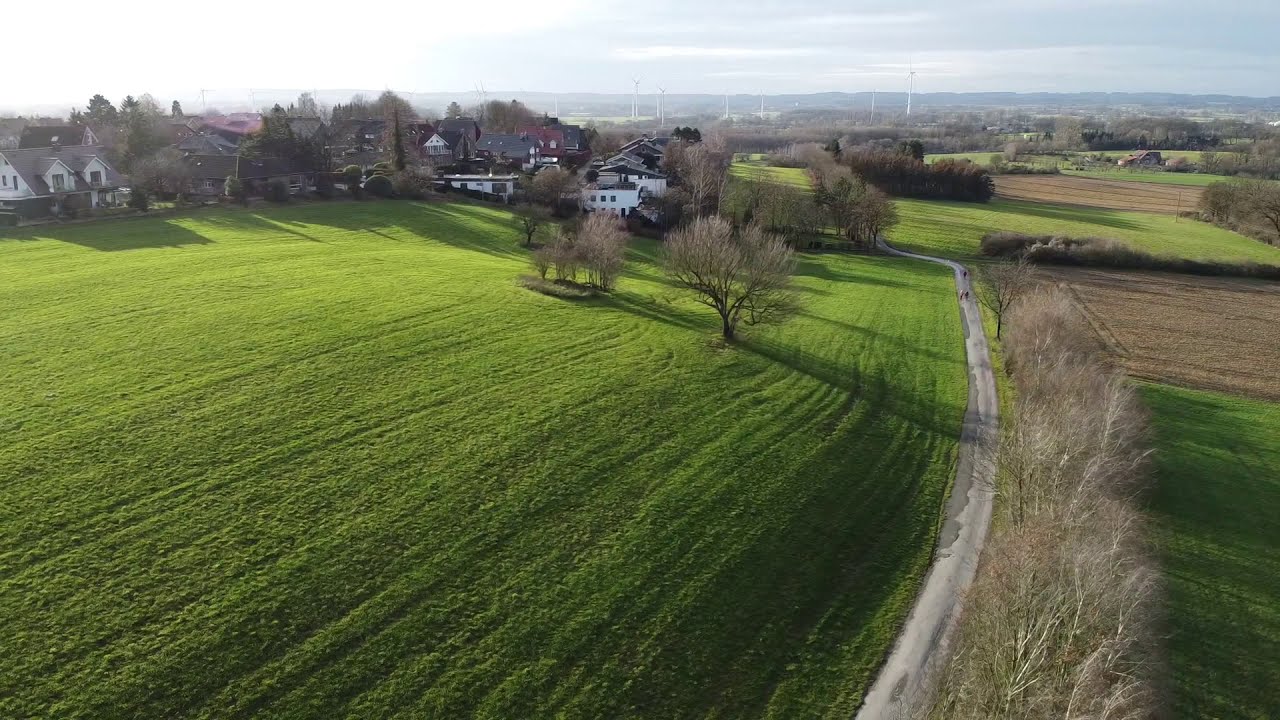The aerial photograph captures a picturesque rural suburban landscape, predominantly featuring a vast, verdant grassy field bathed in sunlight, with accompanying shadows cast by a few scattered trees. To the right of the image, a dirt road runs vertically, flanked by well-maintained leafless trees. The top left of the image reveals a small town with large two-story houses, notably a white house with an A-frame black roof, among other similar white houses with black roofs. In the background, a horizon line showcases small hills or a mountain range under a sky dotted with gray clouds. Windmills dot the fields, adding a distinctly European touch to the scene. Additionally, an asphalt one-lane road with three people walking on it traverses between the grassy field and the brown tilled dirt patches, completing this serene and expansive drone-captured landscape.